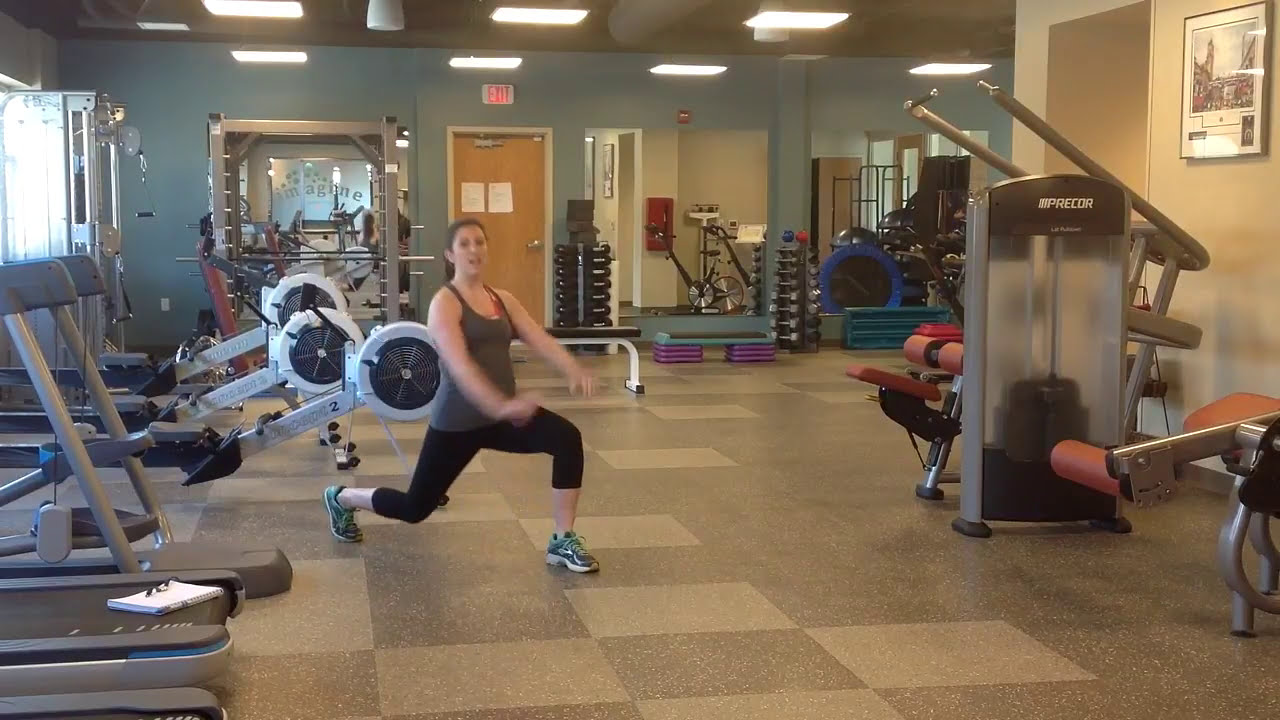In this well-lit gym with blue and white walls, a woman is captured mid-lunge, her form focused and determined. She's dressed in black workout pants that reach her mid-calves, a gray tank top, and green sneakers with white soles. Her brown hair is pulled back into a ponytail, and she's looking toward the camera with her mouth slightly open, likely exhaling during her exercise. 

The gym, which appears to be small, possibly tied to a hotel or apartment complex, has a variety of equipment. Gray treadmills are positioned to her left, with a couple of rowing machines behind her. To her right, there’s an assortment of gym gear including a step-up platform, dumbbells, and additional weight machines. The back wall holds a mirror inscribed with the word "Imagine", reflecting a well-organized rack of weights. 

Other details in the room include mirrored walls, bright ceiling lights, and checkered gray and white tile flooring. A brown door marked with a white and red exit sign and two white pieces of paper adds to the background, while a large mirror to the right of the door magnifies the space. Additional equipment like exercise bikes and arm workout machines are dispersed throughout, making the space comprehensive for various workout routines.